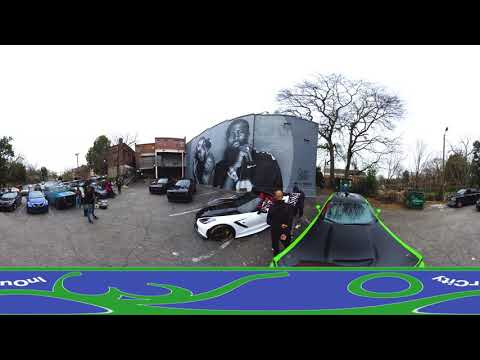The image captures a lively meetup in a parking lot, featuring an array of sleek, high-end cars, primarily matte black sports cars, one with a neon green trim and another with white sides and a black hood and roof. Prominently, there's a large mural painted on a gray, two-story building wall, displaying a black and white depiction of a black man, a white woman, and a child, possibly Kanye West. Adjacent to this building, on the left, is another structure which appears to be apartments. A mix of black and blue cars are scattered throughout the lot, with several people gathered around, all facing away from the camera as they admire the vehicles. In the background, there's a tree extending above the mural's building, adding a touch of greenery to the urban scene. Near the bottom of the image, a dark blue and green banner with squiggly lines and a circle hints at an event taking place in the city, contributing a sense of organized gathering.